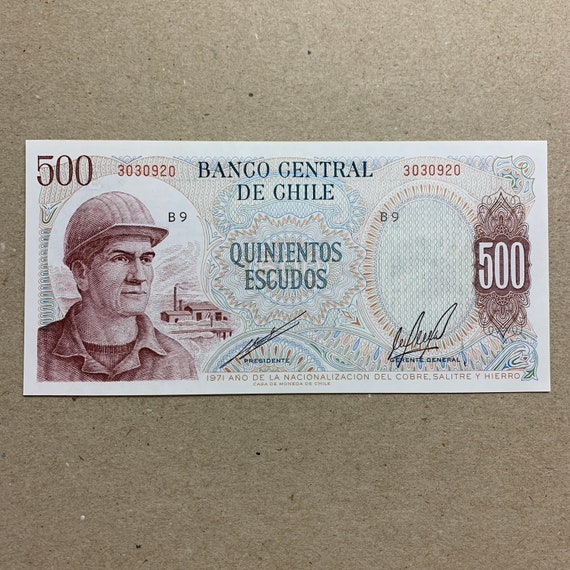This image showcases a piece of Chilean currency, specifically a 500-Quinientos Escudos bill, issued by the Banco Central de Chile. The prominent "500" denomination is displayed in the top left corner and again on the right side, against a henna-styled backdrop. The backdrop of the bill appears to resemble recycled paper or cardboard, giving it a unique texture. In the center, "Banco Central de Chile" is prominently displayed, and beneath it, the value "Quinientos Escudos" is written. The bill features a serial number "3030920" near the 500 mark on the right side, and another seven-digit number next to the 500 on the left. Below much of the imagery, the year "1971" is visible. The bill also contains red and blue elements and includes the signature of the president. To the left side of the bill is an image of a man wearing a hard hat, possibly a construction worker, depicted in a bronzish, brownish-red color.